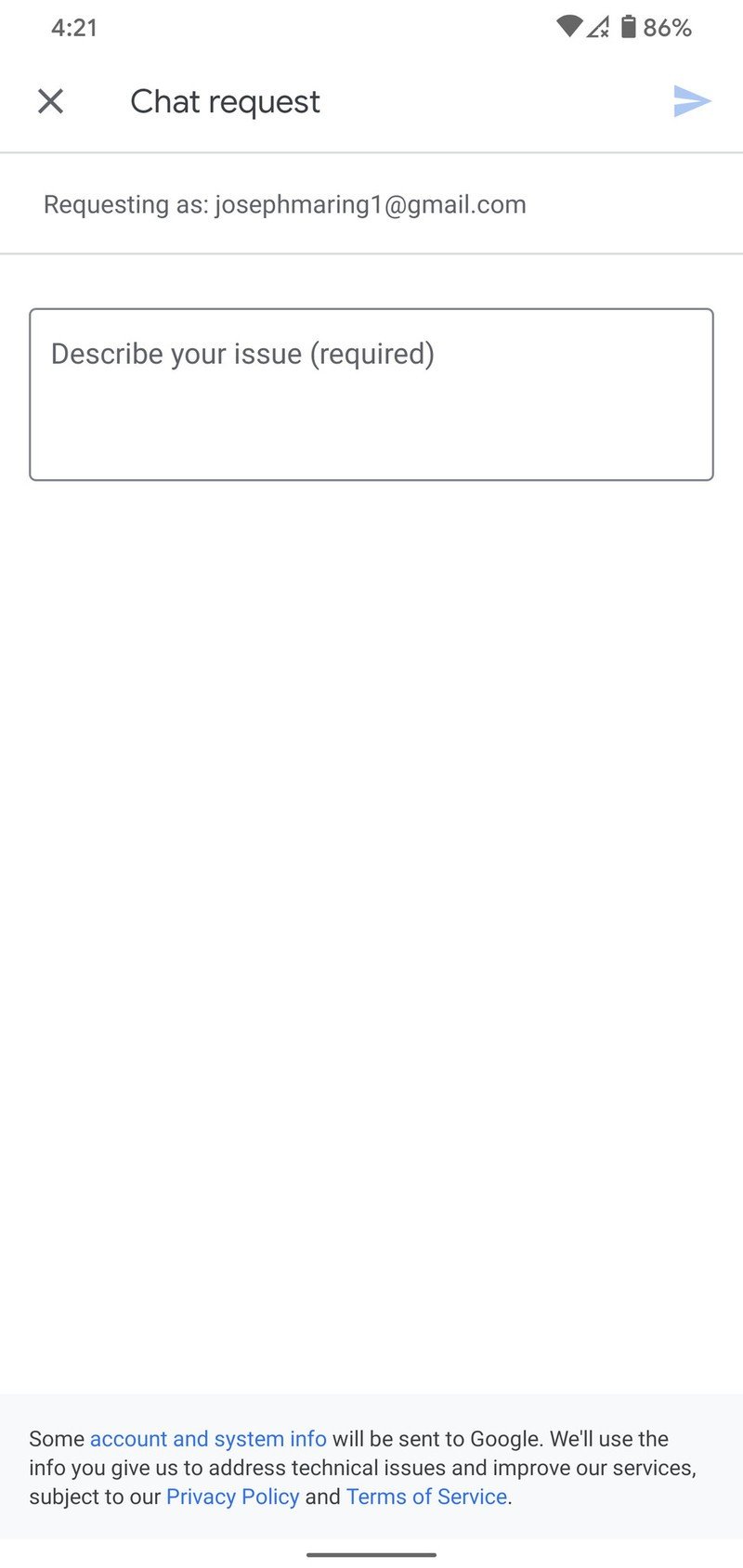This image, captured on a smartphone, depicts a technical support chat interface with the following details:

- **Phone Status**: The phone battery level is displayed at 86%, and a strong network connection is indicated. The current time is 4:21.

- **Chat Interface**: The top section shows a chat request notification with an 'X' icon on the left side, which likely allows the user to close the request, and a blue arrow pointing to the right side, suggesting a progression to the next step in the chat process. The text "requesting as" is shown, followed by the email address "josephmaring1@gmail.com".

- **Issue Description**: Below the email is a gray text box labeled "Describe your issue" with a note "(required)", prompting the user to provide details about their concern. This box offers sufficient space for the user to outline the specific problem they need assistance with.

- **Page Background**: The primary color of the page is white, providing a clean and uncluttered backdrop for the content.

- **Footer Information**: At the bottom of the page, another gray box includes important information starting with "Some account and system info," highlighted in blue, notifying the user that diagnostic information will be sent to Google. It further states, "We'll use the info you give us to address technical issues and improve our services," followed by a note on the privacy policy and terms of service, both of which are also highlighted in blue for easy access to those documents.

- **Page Termination**: A dark gray line at the bottom of the phone screen indicates the end of the current page.